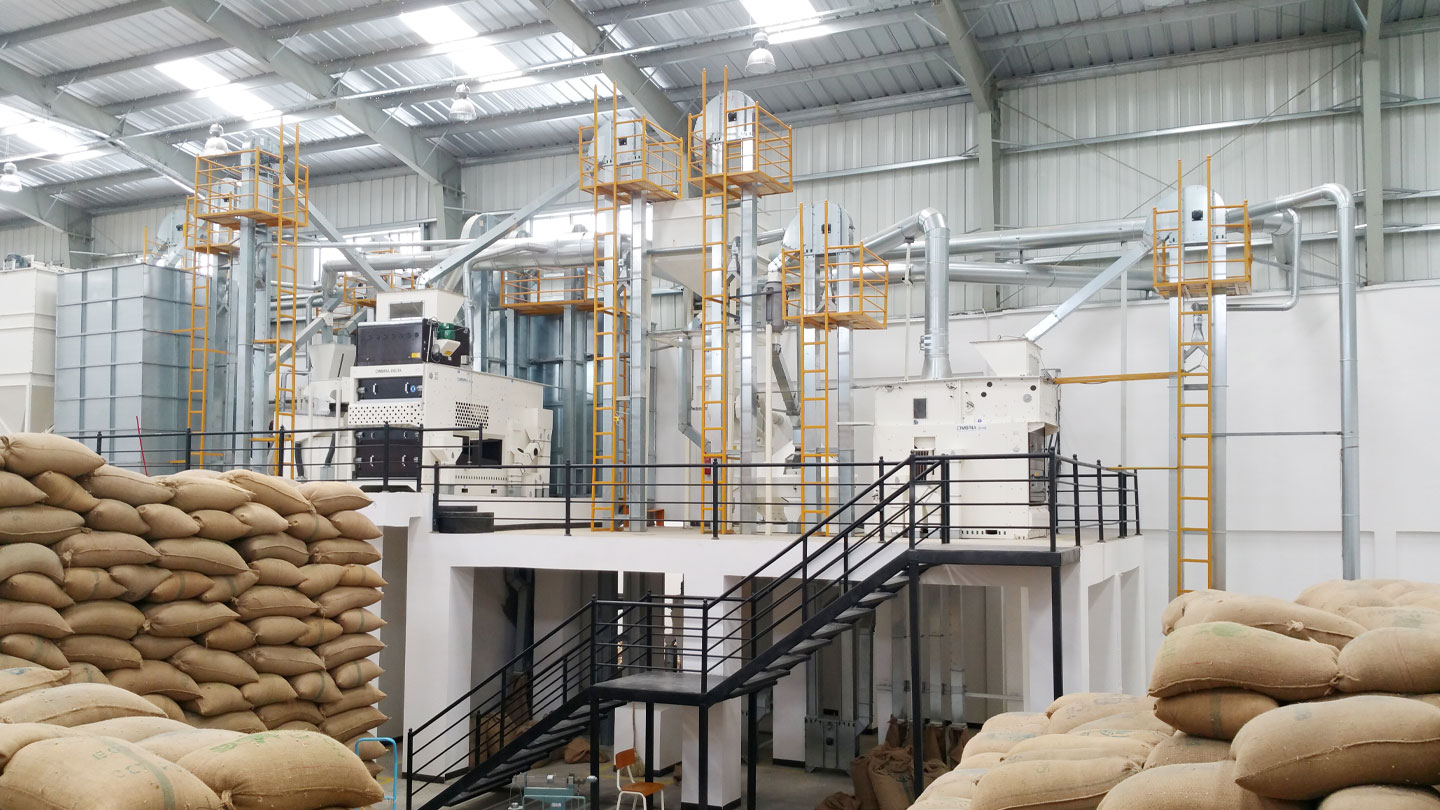The image depicts the interior of a processing plant with bags of an indeterminate brown material, possibly canvas or cement, stacked around the room. The stacks on the left side are particularly high, reaching about 15 layers. The plant is housed within a corrugated metal building supported by metal posts and joists, with fluorescent lights hanging from the ceiling. The complex machinery present includes a white processing machine with control lights positioned in the left center, connected to numerous pipes and tubes of various colors, including yellow, steel, and aluminum. This machinery is arranged across what appears to be a balcony area, accessible via a black steel staircase with a railing. Beneath this balcony, there are small windows, a plastic chair with an orange seat and back, and what looks like a room for people to sit. The ceiling and walls of the facility are primarily white, with the ceiling having a grayish tint.